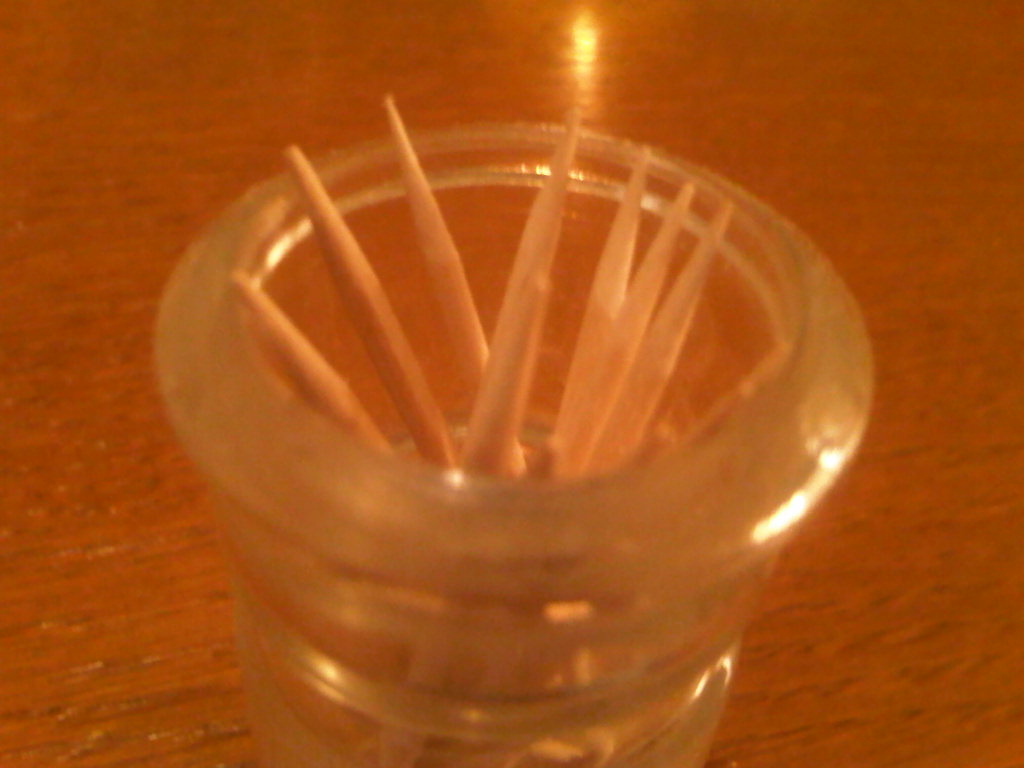This photograph captures a close-up view of an opaque, textured glass container sitting on a medium-to-dark brown woodgrain table with slight marbling and an orange-ish hue. The container, which resembles a shot glass, has a smooth rim and base and is subtly out of focus, contributing to a slight blur, particularly at its bottom. Inside this container are several thick, large toothpick-like items, numbering approximately seven to twelve. Among these, three are distinctly pointed, two have somewhat rounded edges, and the rest are difficult to discern due to the focus and angle of the shot. The image also features a bright yellow glare from an indoor light source near the top-middle right, reflecting slightly off the wooden surface.